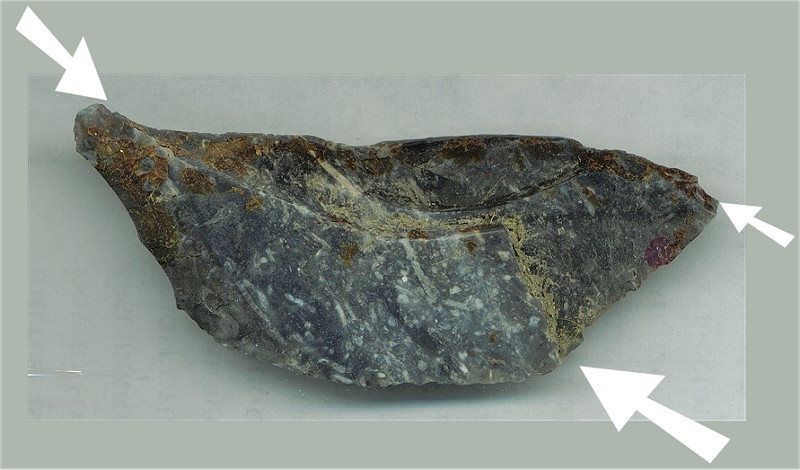The image features a slice of rock characterized by its unique, lip-like shape, with gentle curves on the left and right sides. The rock is displayed on a white surface. Three white arrows are overlaid, highlighting different areas where veins of gold are visible. The rock's core is primarily a deep gray, speckled with white spots, while the right side transitions to a darker gray with distinct purple and brownish residues. The left side is similarly dark, exhibiting greenish residues. Notably, the arrows mark specific points: the left tail end, the right-hand tip, and a light mossy green seam line on the right. This detailed image, replete with annotations, serves as an educational tool, likely for a geology class, illustrating how gold or other materials become embedded within rocks and form intricate veins.